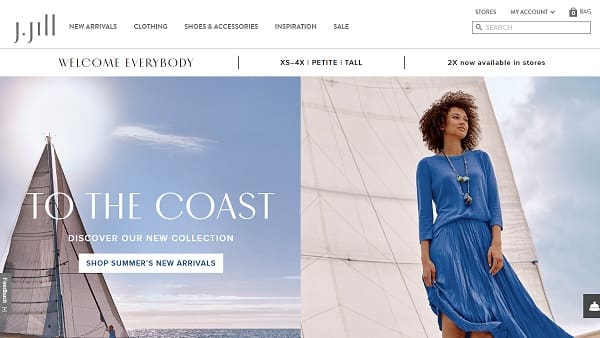A detailed caption for the image described:

---

The homepage of JJill.com captures a serene summer vibe, evoking a sense of stylish discovery. The navigation bar located at the top of the web page offers visitors easy access to various sections such as New Arrivals, Clothing, Shoes, Accessories, Inspiration, and Sale. On the upper right corner, options to locate stores, access personal accounts, and a drop-down menu are available, along with a shopping bag icon representing the user's cart and a search box.

Welcoming viewers with a vibrant message, the site highlights the availability of extended sizes (X4-4X petite call and 2X), now in stores. Dominating the left side of the page, an evocative photograph features a sailboat gently gliding across the ocean with the sun setting in the background, accompanied by text encouraging visitors to "Discover our new collections" and "Shop summer's new arrivals."

Adjacent to this imagery is a striking close-up of a stylish Black woman on the sailboat. She is adorned with a tribal necklace and wearing a flowing blue summer dress, embodying the essence of the season's fashion. Additionally, a small notification bell icon resides at the bottom right, ready to alert customers of updates or messages.

---

This caption intricately details the layout and elements present on the webpage, painting a vivid picture for the reader.